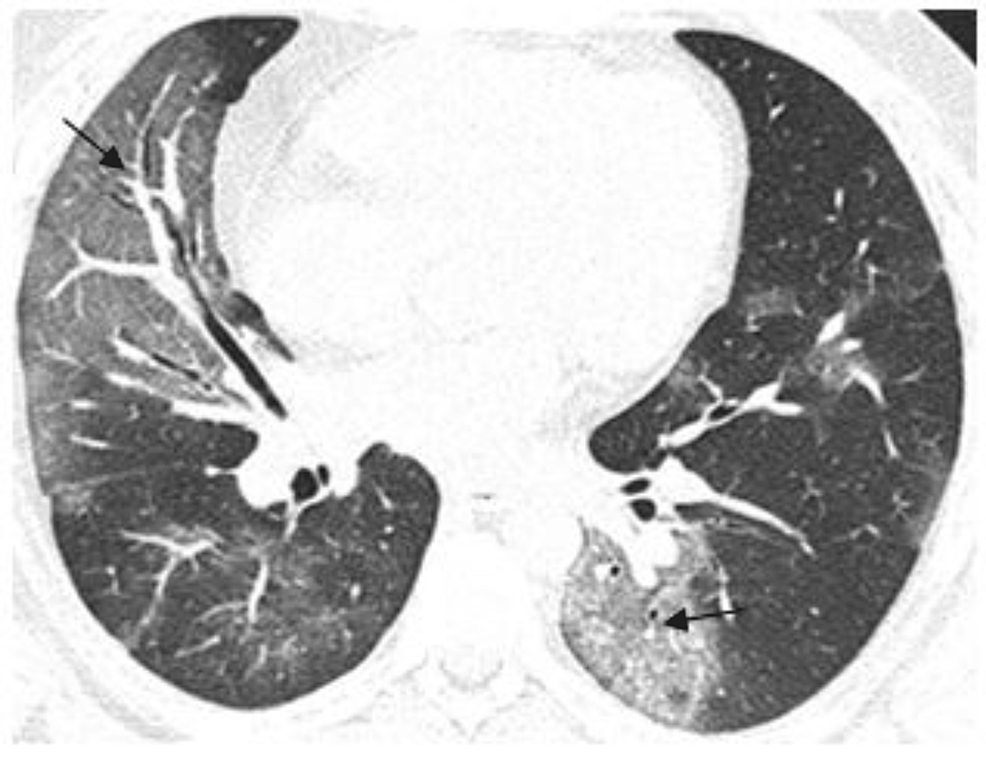The image is a black-and-white x-ray of a pair of lungs. The lungs are prominently displayed on the left and right sides, appearing dark with intricate white tendrils, possibly representing veins or bronchioles, running through them. In the middle of the image is a large, round, white structure dominating the central space. This central shape has two stems extending from it. There are two notable arrows in the image: one in the top left corner pointing towards a structure within the lung, and another in the bottom right corner pointing right at a prominent spot. Additionally, there are two small dots in the bottom left corner of the x-ray.